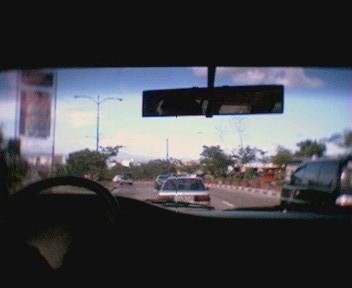A detailed caption for this image could be:

"Captured from the driver's side of a car, this image provides a view through the windshield, from an angle where the person seems to be slightly leaning back. The car's interior is prominently featured, with the steering wheel positioned in the lower left part of the frame and the dashboard extending from the lower left to the lower right. The scene outside the car reveals a highway setting, with two visible lanes. The car is traveling in the left lane while a black van is passing on the right. The rearview mirror is also visible at the upper section of the image, along with part of the vehicle's roof."